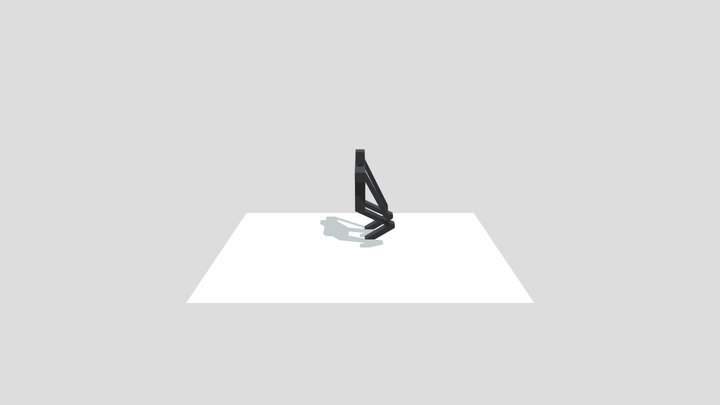This digital image features a black metal structure resembling a person halfway between kneeling and standing, viewed against a white piece of binder or typing paper with a light blue-gray background. The structure lacks a distinct neck, and instead, a knob appears on top, giving it a large stick figure-like appearance. It has shoulders that transition into a vertical torso and then two bent shapes at what could be considered knees. The legs extend downwards from the knees to where the object meets the paper surface. The arms, straight and positioned as if they are touching the knees, complete the human-like form. The figure casts a shadow, which further delineates its form, emphasizing its all-black color with subtle gray outlines.